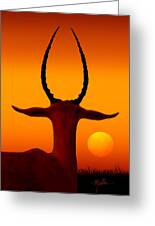This digital mock-up of a possible greeting card features an artistic rendering of a gazelle, or an unusual antelope, set against a strikingly vivid orange sunset. The central focus is a rear view of the gazelle, revealing its long neck, partially visible body, and ears pointing out to the left and right. Rising prominently from its head are U-shaped horns, nearly meeting at their peaks and extending upward with a slight curve. Situated near the gazelle is a large, round, dark orange sun, positioned just above the horizon. The scenery below, likely representing the African plains, is depicted in dark, almost black hues, creating a contrasting silhouette effect against the bright, sunset sky. The card, which appears semi-open and standing, shows some blurriness, further emphasizing the artistic rather than photographic nature of the image.